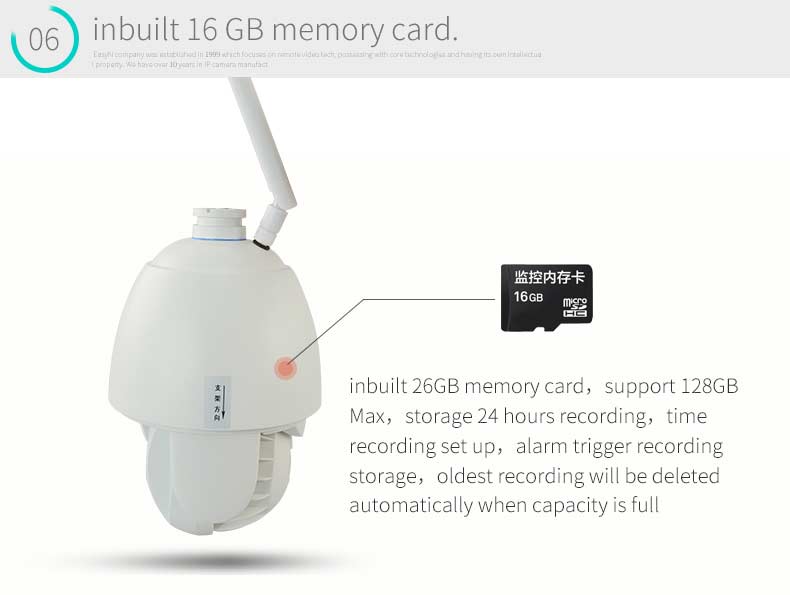This image captures a section of a webpage primarily featuring a pale white and gray color scheme. At the top of the page, a gray rectangular bar prominently displays the text "Inbuilt 16 GB memory card." Below this bar, there is additional gray text, though it is not legible in the image. To the left of the text, a turquoise circle is partially open at the upper left and contains the number "06."

Further down, the image displays a white object adorned with Asian characters and an English description beside it. The English text reads: "Inbuilt 26 GB memory card, supports 128 GB max. Storage for 24 hours recording, time recording setup, alarm trigger recording storage. Oldest recording will be deleted automatically when capacity is full." Adjacent to this descriptive text, there is a picture of the actual memory card, which is black in color.